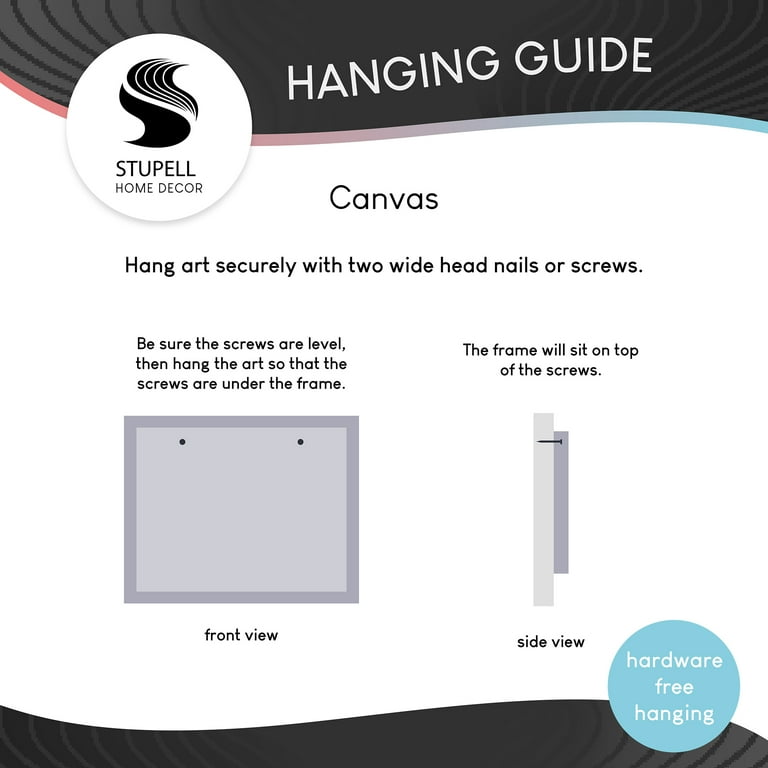This image is a professionally designed "Hanging Guide" by Stupel Home Decor. At the very top, the large and bold title reads "Hanging Guide." On the top left corner, the Stupel Home Decor logo appears alongside the phrase "Build Home Decor." 

The central section of the guide prominently features the word "Canvas" and provides detailed instructions, stating: "Hang art securely with two white head nails or screws." Accompanying these instructions are clear visual aids: 

1. On the left side, there is a front view illustration demonstrating how to ensure the screws are level. 
2. On the right side, a side view illustration shows the frame sitting securely on top of the screws. The caption advises, "Be sure the screws are level, then hang the art so that the screws are under the frame," emphasizing that "the frame will sit on top of the screws."

Additionally, in the bottom right corner, a blue circle with white text declares "Hardware-Free Hanging" against a black wave design. The background of the poster features subtle colors, including light violet, gray, and black, adding a modern aesthetic akin to early 2000s PowerPoint graphics.